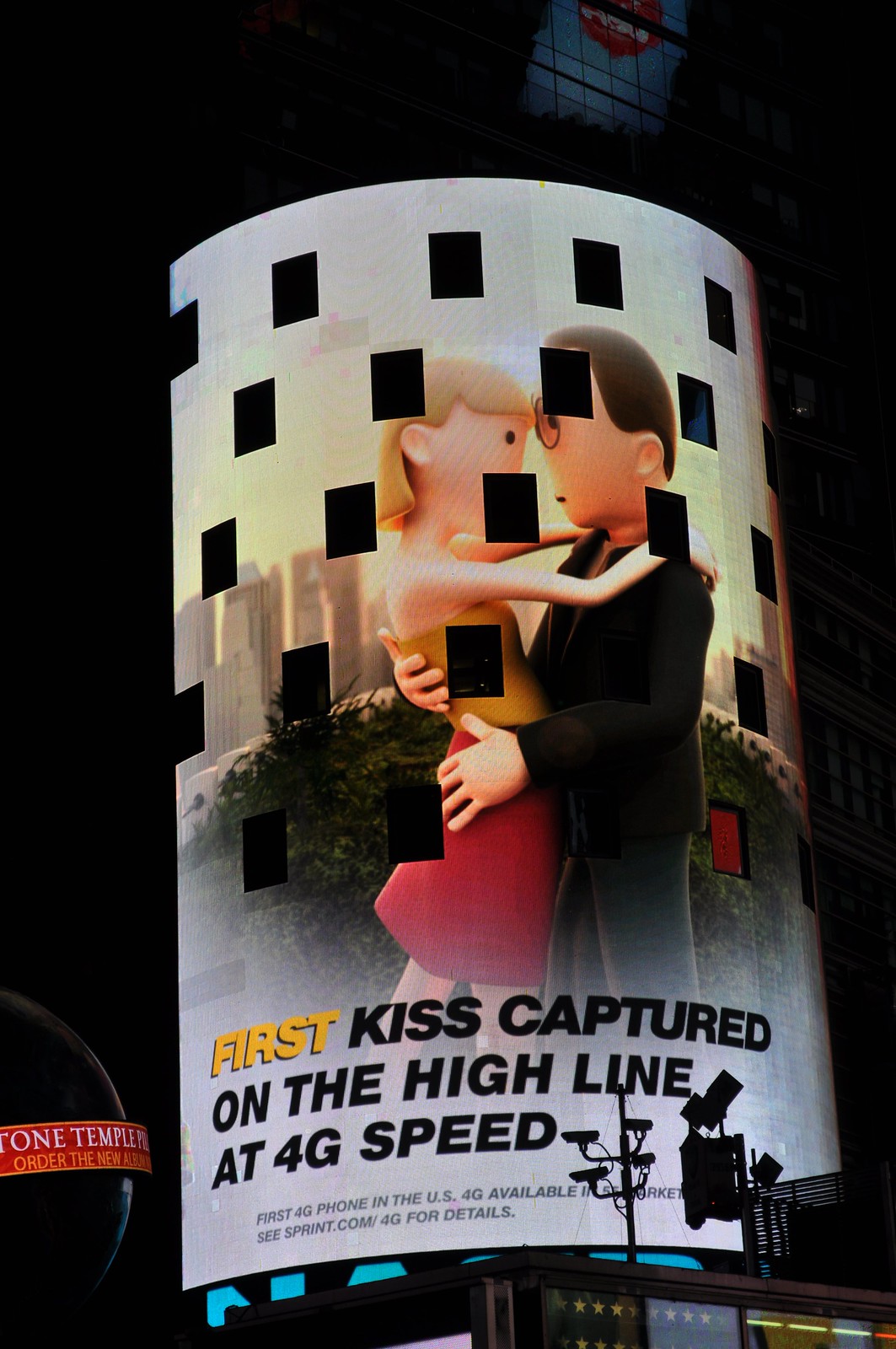This is a nighttime photograph of a large, circular tubular-shaped billboard situated in an area reminiscent of Times Square. The billboard features an animated claymation image of a Caucasian couple engaged in a tender embrace. The woman, with blonde hair and pale skin, gazes into the eyes of the man as she wraps her arms over his shoulders. She is attired in a yellow dress that transitions to a red skirt, revealing her pale legs. The man, with brown hair and glasses, is dressed in a dark coat and has his hands around the woman's waist and rump. Below the couple, the text on the billboard reads: "First" in yellow font, followed by "kiss captured on the High Line at 4G speed" in black font. The night sky frames the billboard from the upper left and right, emphasizing the illuminated display.